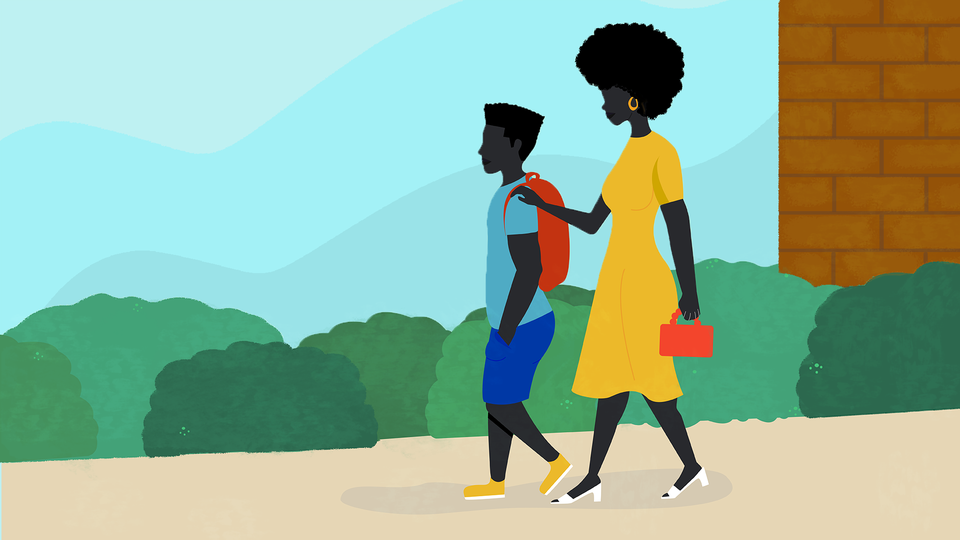In this digital drawing, we see a mother and her presumably young son, both of African descent, walking together. The scene captures their journey away from a brick building, bathed in a simplistic and cohesive color palette. The mother, sporting a tall afro, wears a long yellow dress, complemented by yellow hoop earrings, white mid-heel flats, and carries an orange-red purse. The son, adorned with a flat top hairstyle, is depicted in a blue t-shirt, dark blue shorts, yellow shoes, and a red backpack. Their profiles are notable, with minimal facial details rendered except for the shading of the mother's lips in black. The composition includes green bushes and a hint of sky and mountains in the backdrop, enhancing the pastoral atmosphere. Both figures are centrally placed, walking leftward across a dirt path, highlighting their movement and connection.